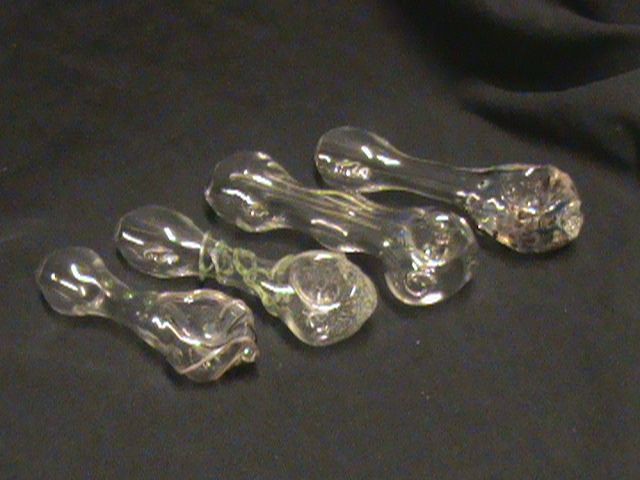This image depicts four small glass smoking pipes arranged on a black fabric, progressing in size from the smallest on the left to the largest on the right. The black cloth underneath them is slightly wrinkled, particularly noticeable in the upper right corner, which adds a textured backdrop to the scene. Each pipe is crafted from clear, see-through glass and features distinctive design elements within the glass itself. 

Starting from the left, the smallest pipe has delicate blue and red colored spots embedded inside. The second pipe appears mostly plain but is adorned with three or four gold streaks. The third pipe, which is slightly larger, has a wrapping of what looks like a gold string around it, and the fourth and largest pipe has minimal decoration, characterized by its simplicity. There are subtle lines of green and yellow running vertically within the glass of some pipes.

Each pipe is shaped somewhat like an hourglass, with a small indentation at the top for the bowl, which is where tobacco or another substance can be placed. The pipes also feature a bulbous end and a cylindrical middle section. Despite the picture being a bit blurry and grainy, the reflective quality of the glass causes the items to shine, capturing the light effectively and enhancing the visibility of the internal designs and decorations.